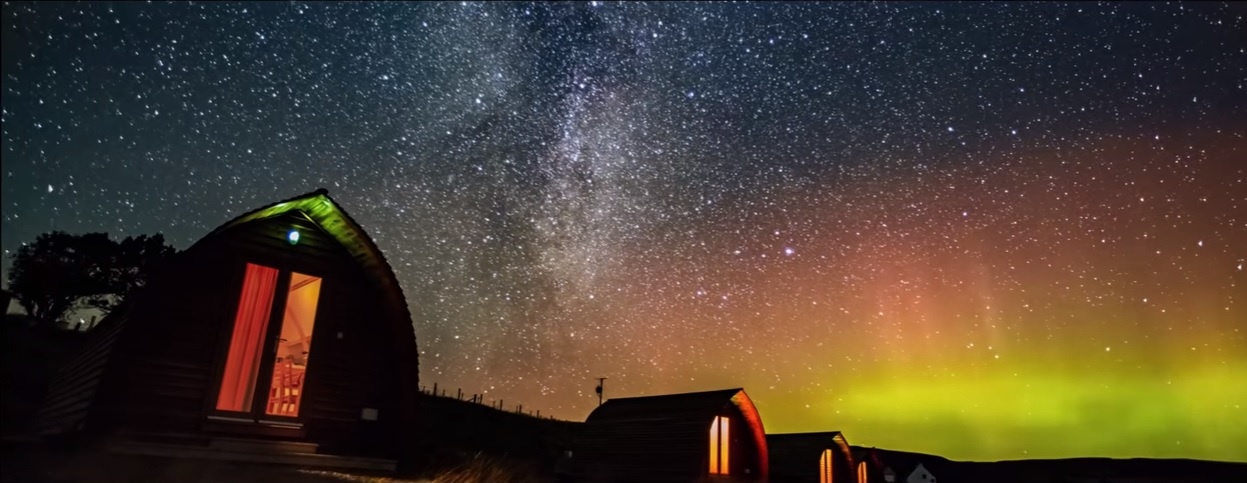In this panoramic night sky photograph, thousands of stars illuminate a clear, pollution-free space. The vast, star-studded sky transitions from black to vibrant hues of orange, deep yellow, and green on the right, suggesting an auroral effect. The ground is dotted with small, oval-shaped buildings that resemble sheds or tiny huts, each glowing warmly with lights on inside, sometimes visible through curtained windows. In the leftmost building, orange curtains partially cover the double windows, through which a desk and table can be faintly seen. Above the windows, a small blue light casts a greenish glow inside the triangular part of the building. A solitary antenna-like structure stands on the far right, initially mistaken for a person. In the far left background, a tree completes the serene, starlit landscape.